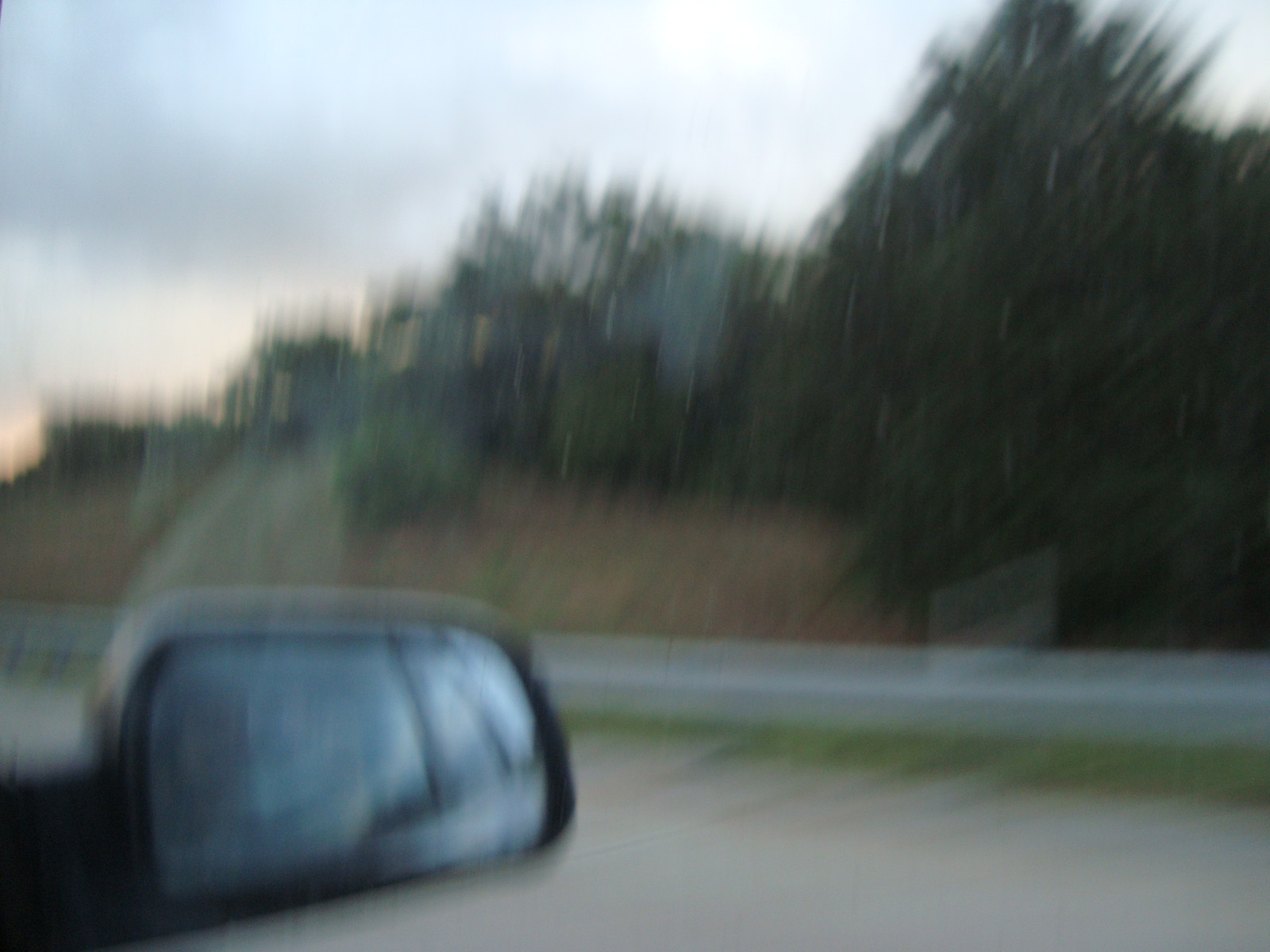In this image, there is a slightly out-of-focus countryside scene featuring a paved road that runs through the middle. On the near side of the road, there is a parked silver car. The road is lined with grass verges on both sides and has a white line running down its center. On the far side of the road, the scene is lush with various trees and bushes, along with a grassy area. A path appears to gradually ascend the slope in the distance, adding depth to the landscape. The sky overhead is cloudy, suggesting an overcast day, and the tops of the bushes are noticeably bent to the right, indicating strong winds.